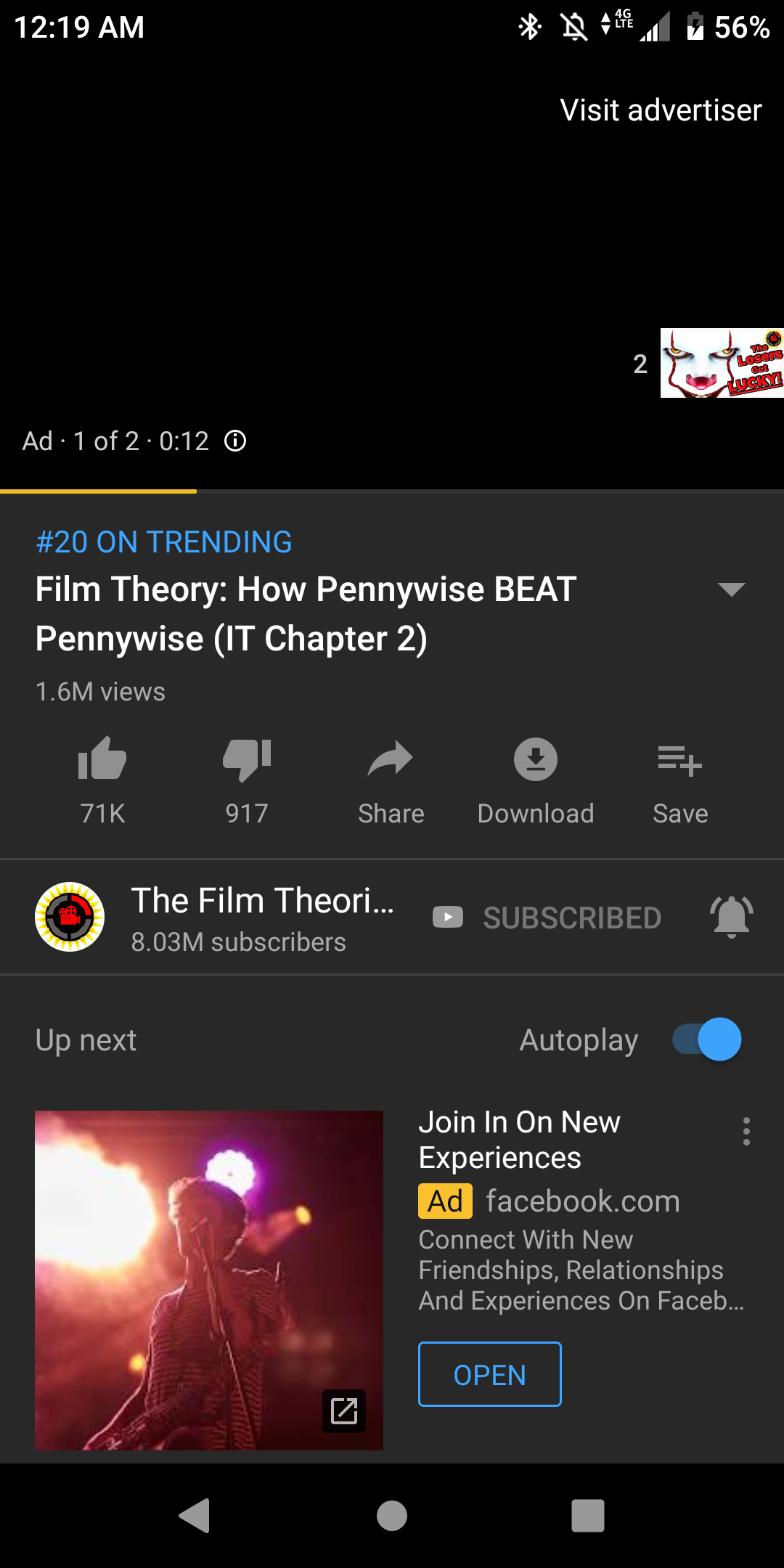The image is a screenshot from a cell phone, with a display approximately three times taller than it is wide. The entire background is black, highlighting the white text and icons. At the top left corner, the time is shown as "12:19 AM." On the upper right, various status icons are visible: the volume is muted, the signal strength is at half capacity, and the battery is at 56%.

Below this top area, the interface appears to be from YouTube. The video space is currently blank, except for the text "Visit Advertiser" in the upper right corner. A countdown timer for skipping the ad is positioned in the lower right corner, showing 2 seconds remaining. In the lower left of the video area, it states "Ad 1 of 2, 12 seconds long." Directly below, a progress bar indicates about 25% completion of the ad.

Further down, in teal text, it mentions "Number 20 on trending". Beneath that, in white text, the video title reads "Film Theory: How Pennywise Beat Pennywise (IT Chapter 2)." Light gray text below the title notes "1.6 million views." Standard YouTube buttons are aligned underneath, including thumbs up (71,000 likes), thumbs down (917 dislikes), share, download, and save options.